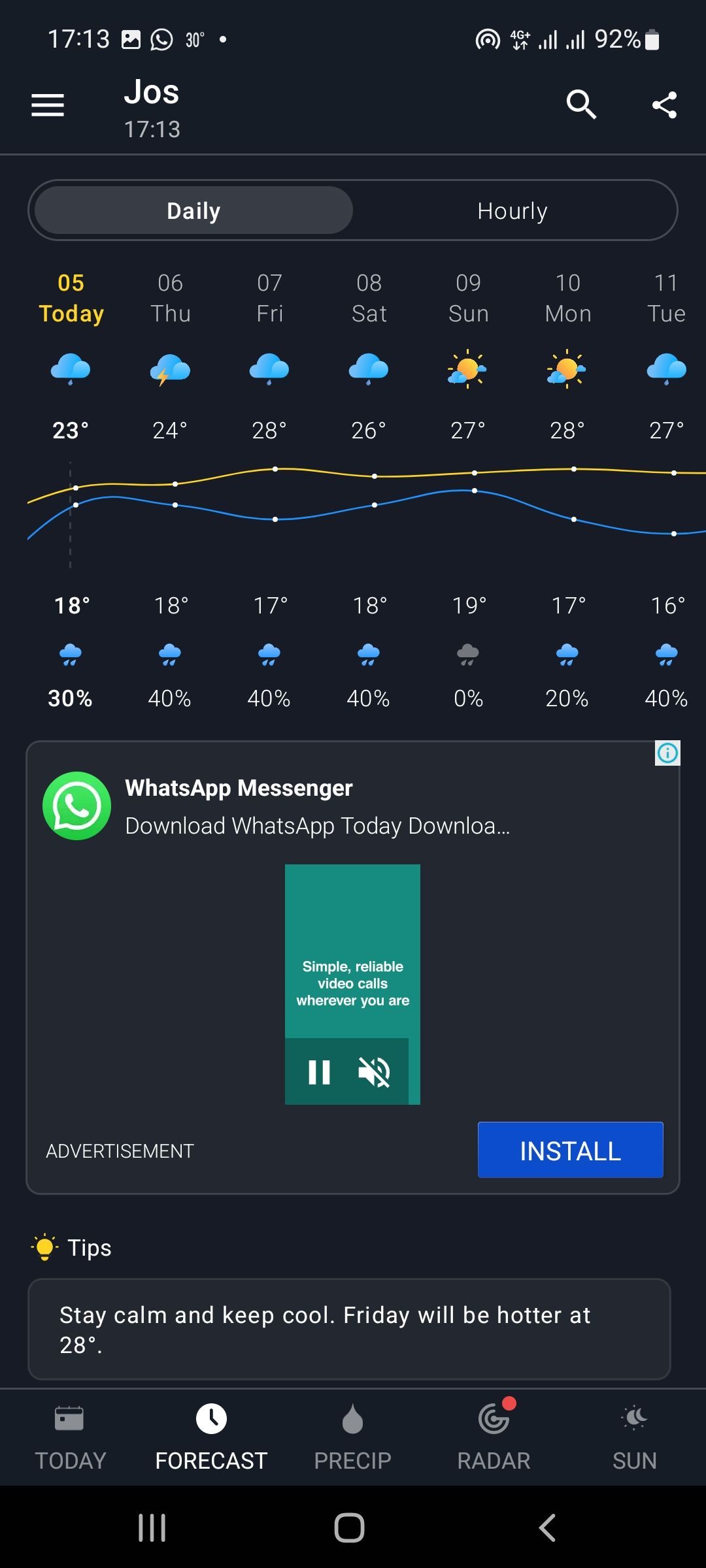The image portrays screenshots of an Android device displaying weather forecasts for the current week, spanning from Wednesday to Tuesday the 11th, specific to the location "Jers." The device's time is shown as 17:13, and visible icons include the gallery, WhatsApp, and an active hotspot indicator. The network signal bars for two SIM cards are both at full strength, and the battery level is at 92%. Additionally, there's an advertisement for WhatsApp Messenger included on the page. The daily temperatures are detailed as follows: 23°C for Wednesday, 24°C for Thursday, 28°C for Friday, and projections continue thereafter.